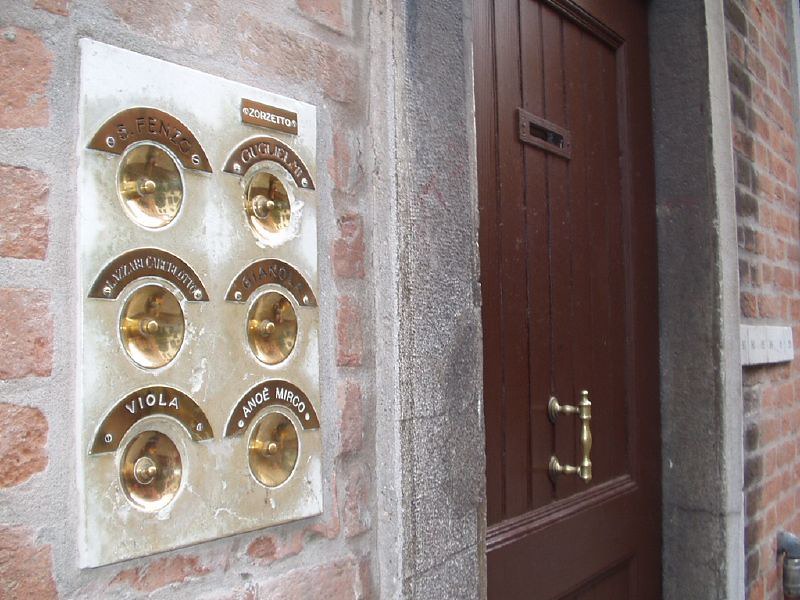The photograph captures an old, rustic red brick building with a weathered appearance, indicative of its age. The large wooden front door, which is brown with a single gold, vertical doorknob centered in the middle, stands prominently within a cement doorway. At the top of the door is a horizontal rectangular slot, likely for peering outside.

To the left of the door, there is a white plate marked with age, featuring six distinct round golden doorbells arranged in two columns of three. Each doorbell is set within a concave structure, accompanied by an arched golden plaque displaying the names of residents—like Viola and El Mirko—in white writing. This unique arrangement of labeled doorbells enhances the historic charm of the building.